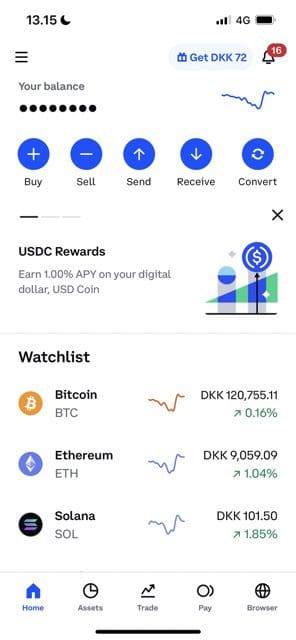"This screenshot from a cell phone displays a stock app interface. At the top left corner, the time is shown as 13:15, next to a moon symbol indicating a night mode setting. Directly below, a message reads 'Get DKK 72,' aligned to the right, followed by a notification icon with the number 16. Further down, there is the text 'Your Balance' aligned to the left, below which is a horizontal row of approximately eight dots, indicating page navigation. To the right of these dots, a blue line, resembling a graph marker, is visible. Beneath this section, there are five buttons labeled 'Buy,' 'Sell,' 'Send,' 'Receive,' and 'Convert.' The last part of the screenshot shows 'USDC Rewards' along with a graph icon and a monetary symbol positioned above it to the right."